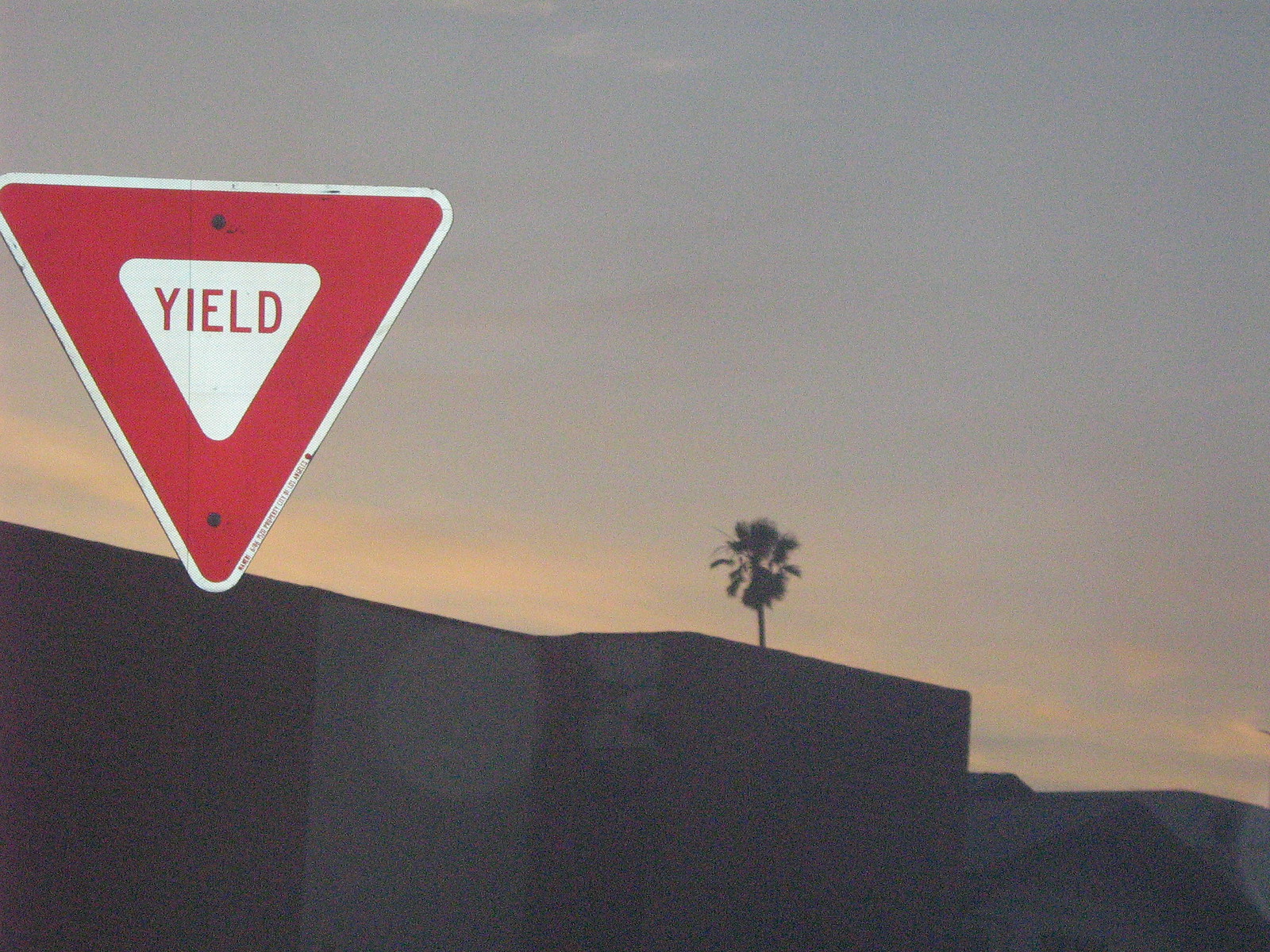The image showcases a yield sign prominently placed against a vibrant blue and grayish sky backdrop. The yield sign, an upside-down inverted triangle, is detailed with a white inner triangle featuring the word "YIELD" in bold red letters. Surrounding this central triangle is a thick red border, further defined by an additional bordering white edge. Noticeable dark bolts are fixed at the top and bottom of the sign, suggesting it is fastened to a pole, although the pole itself is cropped out of the frame. In the foreground, a solitary dark-colored palm tree stands adjacent to a large, boxy man-made structure characterized by its sharp edges and right angles. To the right of this structure, a series of natural, dark-colored hills enhances the composition, creating a juxtaposition between nature and man-made elements. The overall lighting and color tones of the image hint at a slightly overcast atmosphere, enriching the visual contrast.